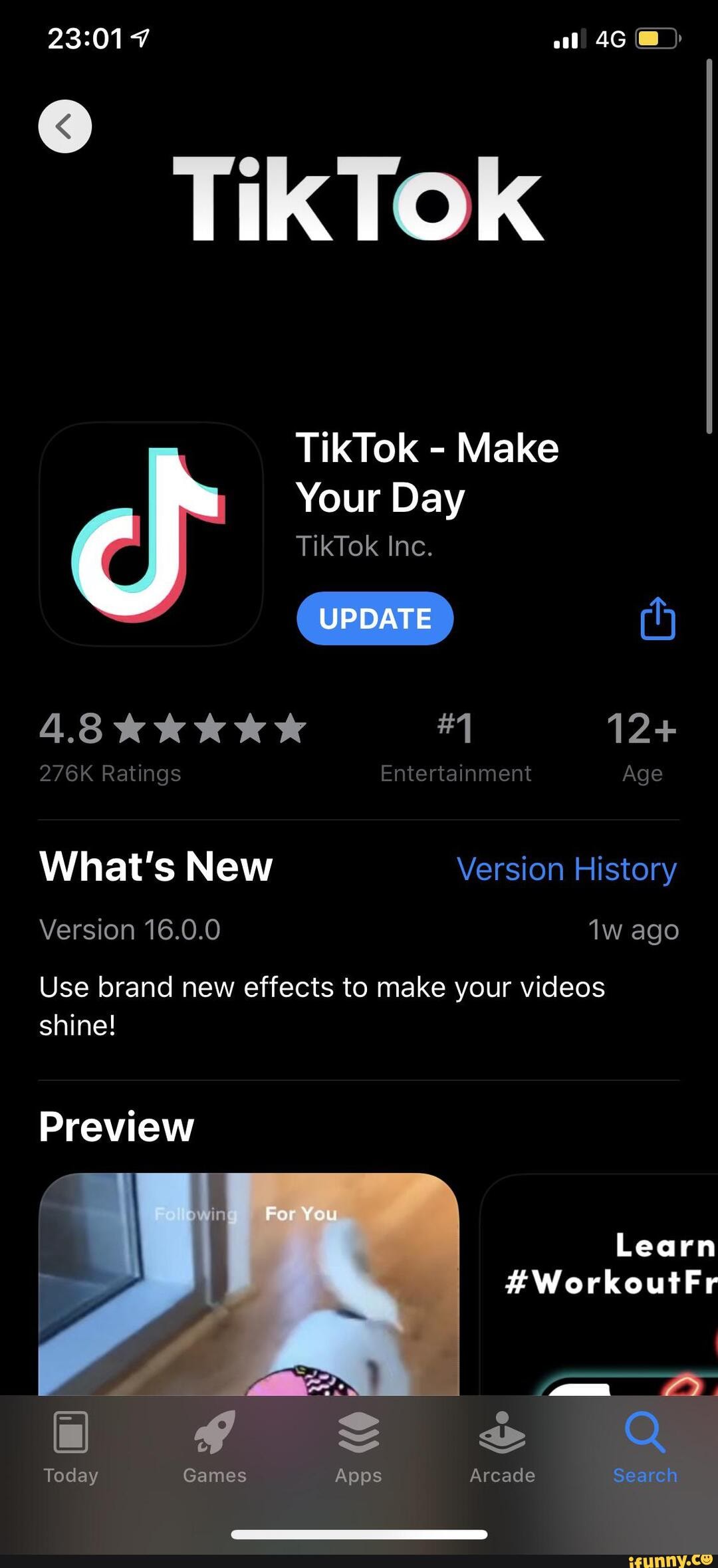The image depicts the TikTok application update screen from an app store, likely viewed on a cell phone or tablet. The background is predominantly black. In the status bar at the top-left corner, the timestamp reads 23:01, while the top-right corner displays three out of four signal bars on a 4G network and a battery icon that is half-filled and yellow. Just below the status bar, in bold lettering, "TikTok" is prominently displayed. 

Below "TikTok," the screen features a gray circular back arrow for navigation. Adjacent to this is the TikTok icon accompanied by the text "TikTok - Make Your Day," followed by "TikTok Inc.," and an "Update" button in a blue tab with white text. TikTok boasts a high rating of 4.8 stars based on 276,000 reviews, is ranked number one in the entertainment category, and is recommended for ages 12 and older (though the user remarks it should be for ages 100 and older).

Underneath these details, a faint gray line demarcates the section that lists new updates with "What's New" in white text, followed by "Version History" in blue text. The latest update mentioned is "Version 16.0.0" which was released one week ago with the notes: "Use brand new effects to make your videos!" Another faint gray line separates this section from a "Preview" section. The preview image below this text features a For You page, prominently showing the back of a white dog, though the rest of the content is not easily discernible.